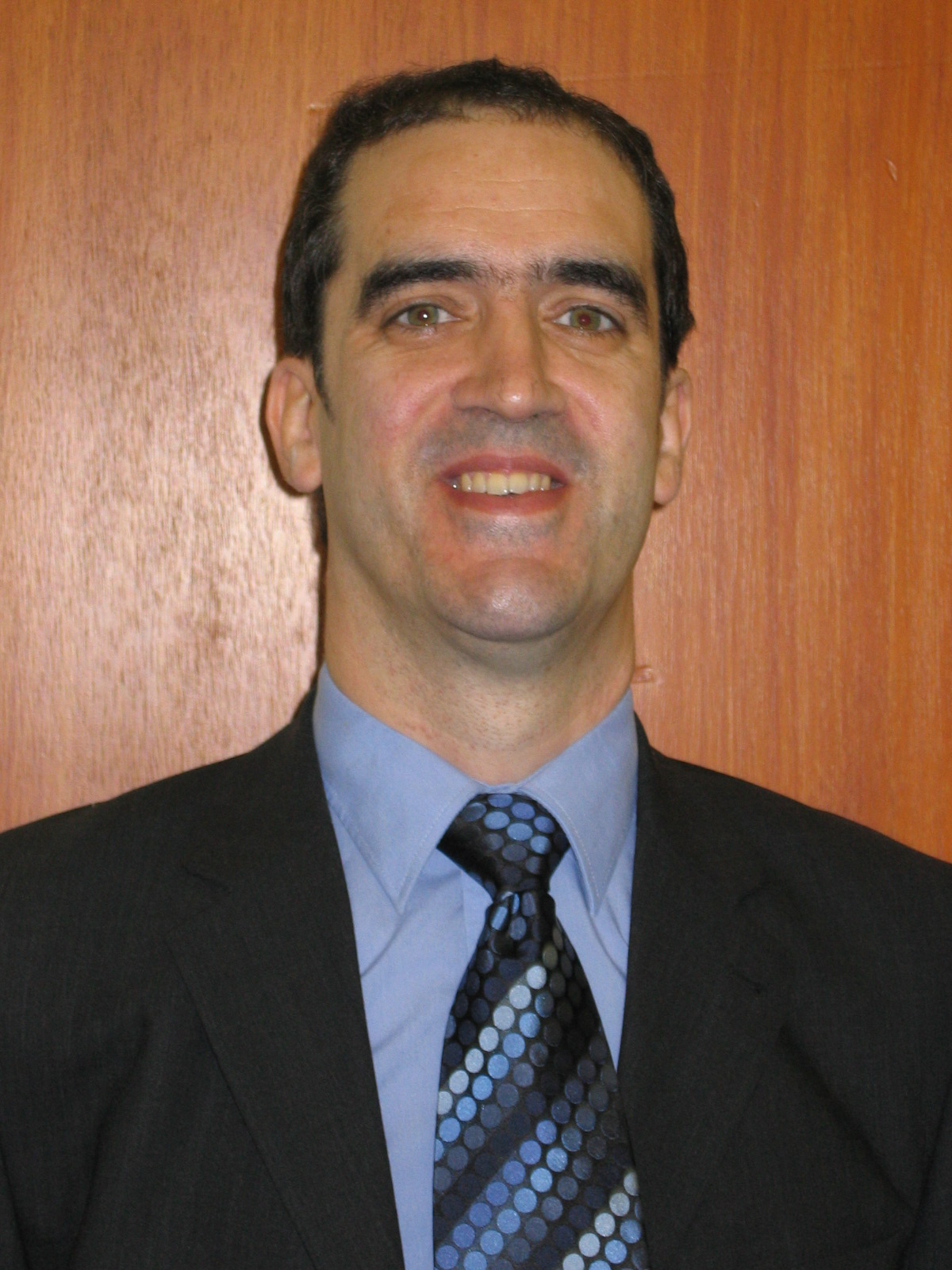In this image, we see a man whose face and bust are prominently displayed. He has a distinct appearance characterized by short, dark, thinning black hair, thick black eyebrows, gray or blue eyes, and a clean-shaven look. His facial features include a small mouth, a pronounced chin, a very long face, and a thick neck. He is smiling warmly and looking directly at the camera. He is dressed in a sophisticated outfit consisting of a black suit jacket, a blue collared shirt, and a striking blue tie adorned with a pattern of light blue, dark blue, black, and gray circles arranged in stripes. The background features a wooden wall or possibly a door with an orange and brown wood grain texture. The overall impression is of a charismatic, possibly familiar figure, impeccably dressed and captured in a moment of amiable composure.